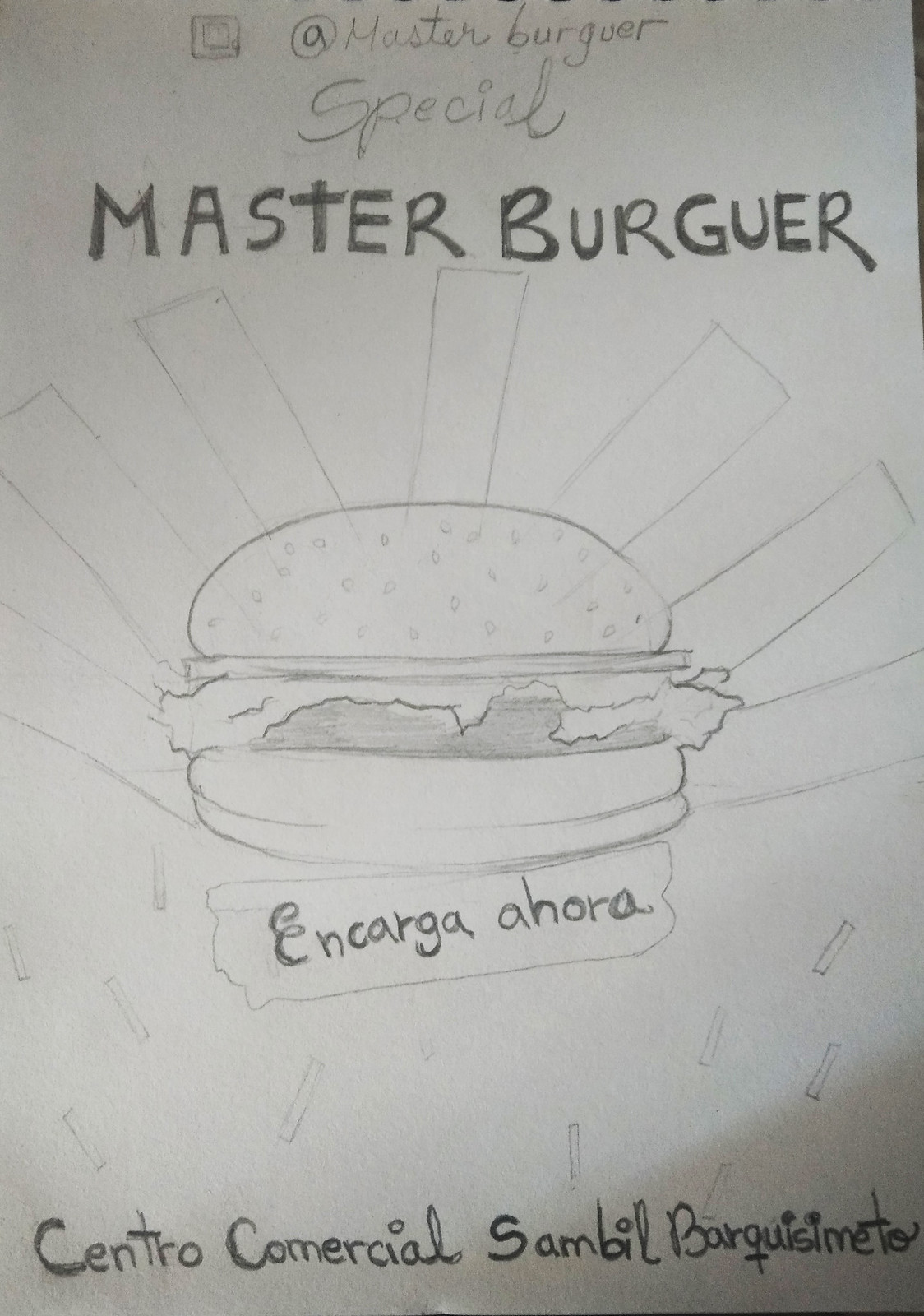This detailed pencil sketch on white paper prominently features a meticulously drawn hamburger on a sesame seed bun at its center. The sesame seeds are represented by small, precise circles. Surrounding the hamburger patty, wavy gray lines skillfully indicate layers of fresh lettuce. Below the bottom bun, within a neatly outlined rectangle, the phrase "Encarga Ahora" is written, translating to "Order Now" in English. At the very bottom of the image, the location "Centro Comercial Sambit Vigresmito" is inscribed. Radiating outward from the hamburger like sun rays, long, thin rectangles arch gracefully from side to side, enhancing the composition. Above the burger, bold lettering created with a marker spells out "Master Burger," while further above, the phrase "Master Burger Special" is lightly sketched in pencil. This artistic representation combines elements of sketching and marker work to create a visually appealing and informative portrayal.